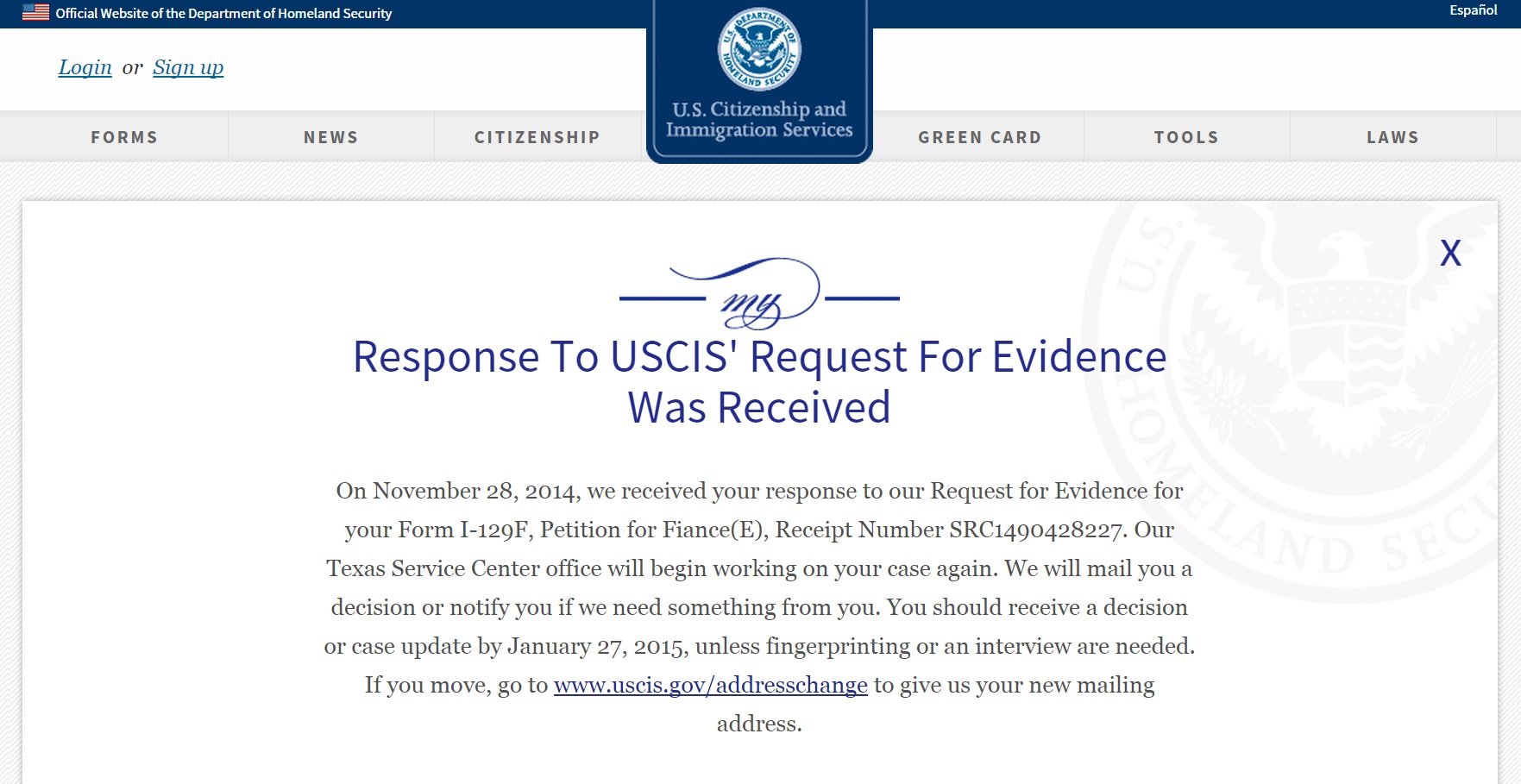A detailed screenshot of the official Department of Homeland Security website, featuring a blue border and an American flag along the top. There is an option for "Español" and buttons to log in or sign up. Prominently displayed in the center is the acronym "USCIS," surrounded by links to various sections such as forms, news, citizenship, green cards, tools, and laws.

The main content of the screenshot is a notification about the processing status of a case. It reads: "My response to the request for evidence was received on November 28th, 2014. We received your response to our request for evidence for your form. I want to petition for financing. The receipt number is SRC 1490428227. Our Texas Service Center will begin working on your case again. We will mail you a decision or notify you if we need something else from you. You should receive a decision or case update by January 27th, 2015, unless fingerprinting or an interview is needed. If you move, you can visit our website to provide your new mailing address."

This appears to be a meticulous capture of the correspondence and status update within an individual's case management section on the official USCIS website.